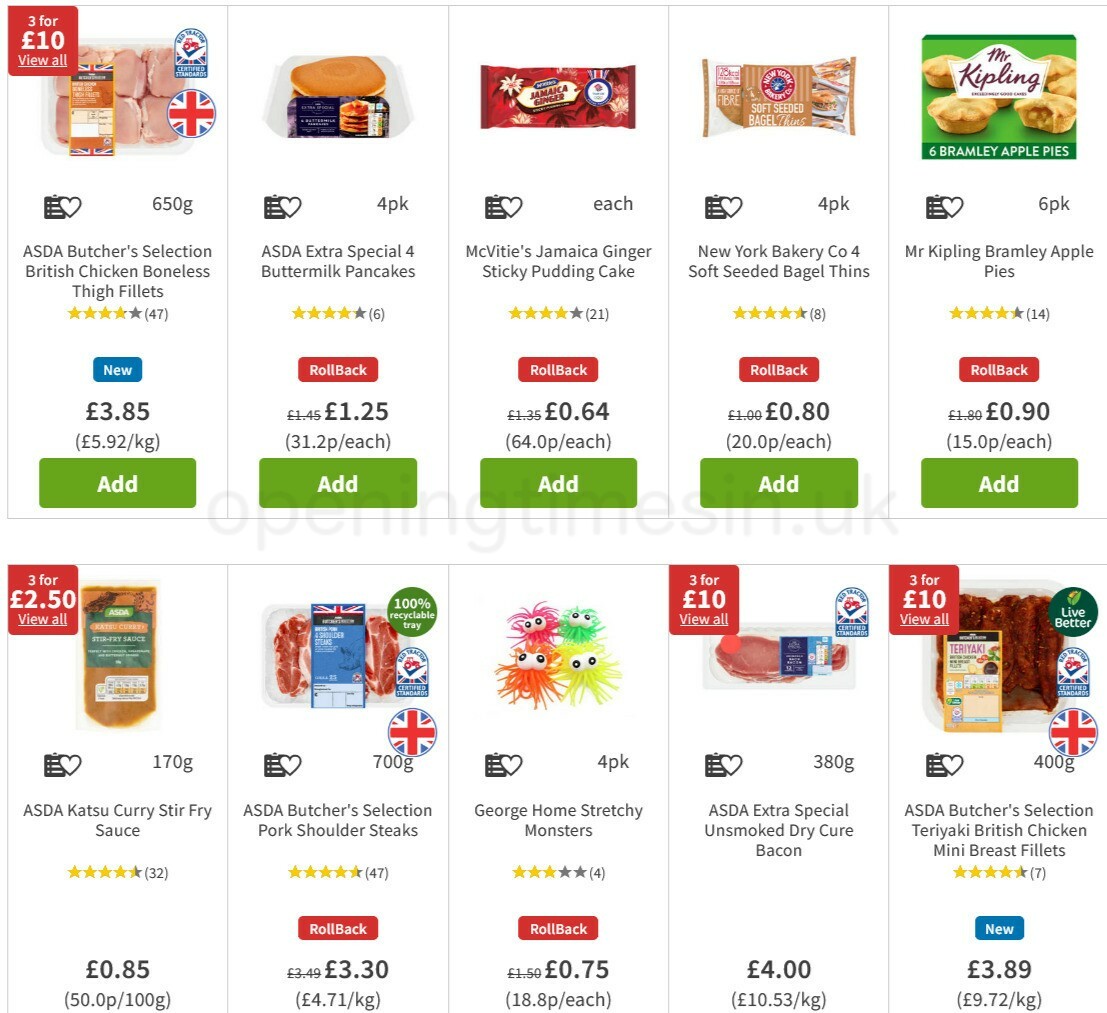The image depicts a webpage designed for online ordering showcasing various grocery items and their prices. Here’s the detailed breakdown of the items listed:

1. **ASDA Butcher Selection British Chicken Boneless Thigh Fillets** - Price: $3.85.
2. **ASDA Extra Special Four Butter Milk Pancakes** - Price: $1.25.
3. **McVitie's Jamaican Ginger Sticky Pudding Cake** - Price: $0.64.
4. **New York Bakery Co. Four Soft Seeded Bagels** - Price: $0.80.
5. **Mr. Kipling Bramley Apple Pies** - Price: $0.90.
6. **ASDA Katsu Curry Stir Fry Sauce** - Price: $0.85.
7. **ASDA Butcher Selection Pork Shoulder Steaks** - Price: $3.30.
8. **George Home Stretchy Monsters (Toy)** - Price: $0.75.
9. **ASDA Extra Special Unsmoked Dry Cured Bacon** - Price: $4.00.
10. **ASDA Butcher Selection Teriyaki British Chicken Mini Breast Fillets** - Price: $3.89.

Each item features an 'Add' button beneath it, enabling easy addition to the shopping cart. The top of the page highlights a promotion stating "3 for 10" with an option to "view all."